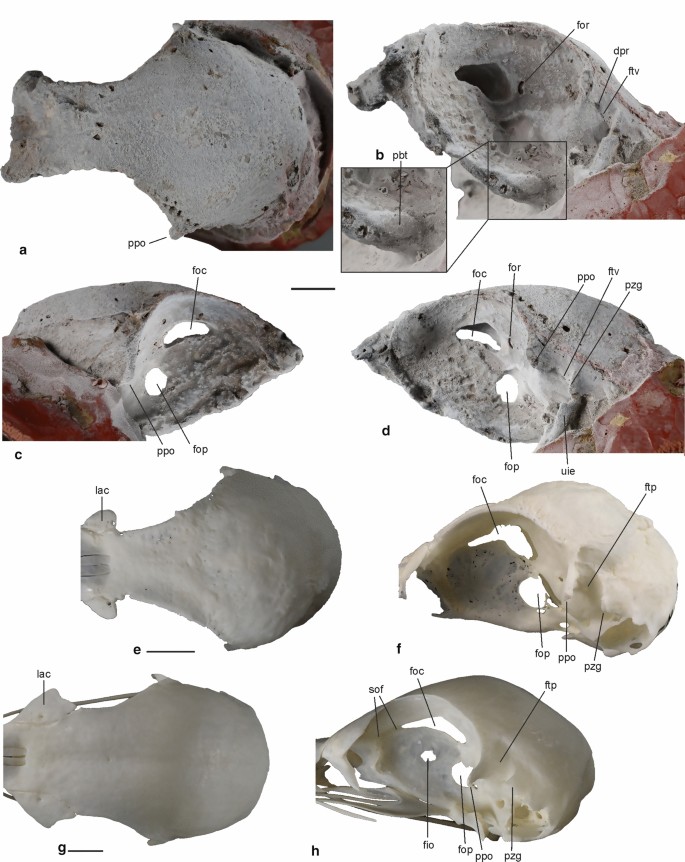The image is a photographic set of eight annotated photos against a white background, showcasing prehistoric tools, possibly cutting instruments or arrowheads. The tools are meticulously labeled with various acronyms. 

- The top photo features a black tool with a blade at the front and a handle-like back, labeled "PPO".
- To the right of it, there's an arrowhead-shaped tool marked "FORDPRTFBV", adjacent to a close-up image annotated "BPBT".
- Below these, an arrowhead with a tapered point and two holes is labeled "FOCFORPPGFTVPPGUIEFOPND".
- Element C mirrors this arrowhead but faces the opposite way and is marked "FPPOFOPFOC".
- Element E appears as a cutter with a semi-circular curved blade and a handle, labeled "LAC".
- Element F, resembling a skull with holes, reads "FOC", "FOP", "PPO", "PZG", and "FTP".
- Element G is similar to Element E but less tapered and also annotated "LAC".
- Finally, Element H, much like Element G but with more holes, displays the letters "SOFFOCFTOFOPPPOPZG" and "FTP".

These tools and elements come together in the last image to suggest a skull, possibly hinting at the reconstruction of a fossil. The acronyms scattered throughout, such as "PPO", "FOC", "FOP", "LAC", and "PZG", remain undefined, adding an element of mystery to the prehistoric assemblage.